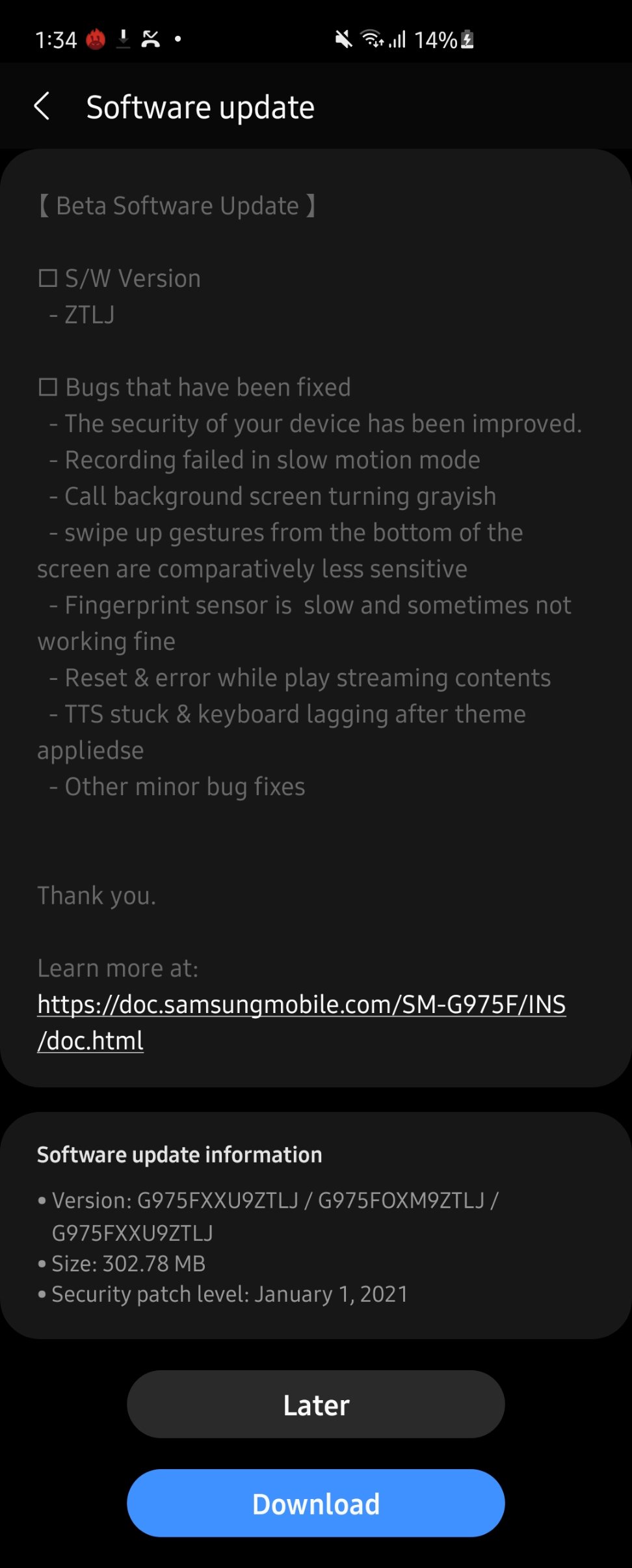The phone screen displays a notification about a software update. The update is identified as a Beta Software Update with the version number "ZTLJ." The notification in white text reads "Software Update," followed by "Beta Software Update" in gray text. The phone shows a range of issues that have been addressed with this update, which includes improvements in device security, fixing the problem of recording failures in slow motion, and resolving a gray screen issue when callback background is activated. Additionally, the sensitivity of swipe-up gestures from the bottom of the screen has been enhanced, the responsiveness of the fingerprint sensor has been improved, and an error while playing streaming content has been corrected. Other minor bugs such as TTS struck and keyboard lag after applying themes have also been fixed. At the bottom, there is a URL for further information: https://doc.samsungmobile.com/sm-g975f/ins/doc.html. The phone screen also indicates 14% battery life, a missed call, and the sound being turned off.